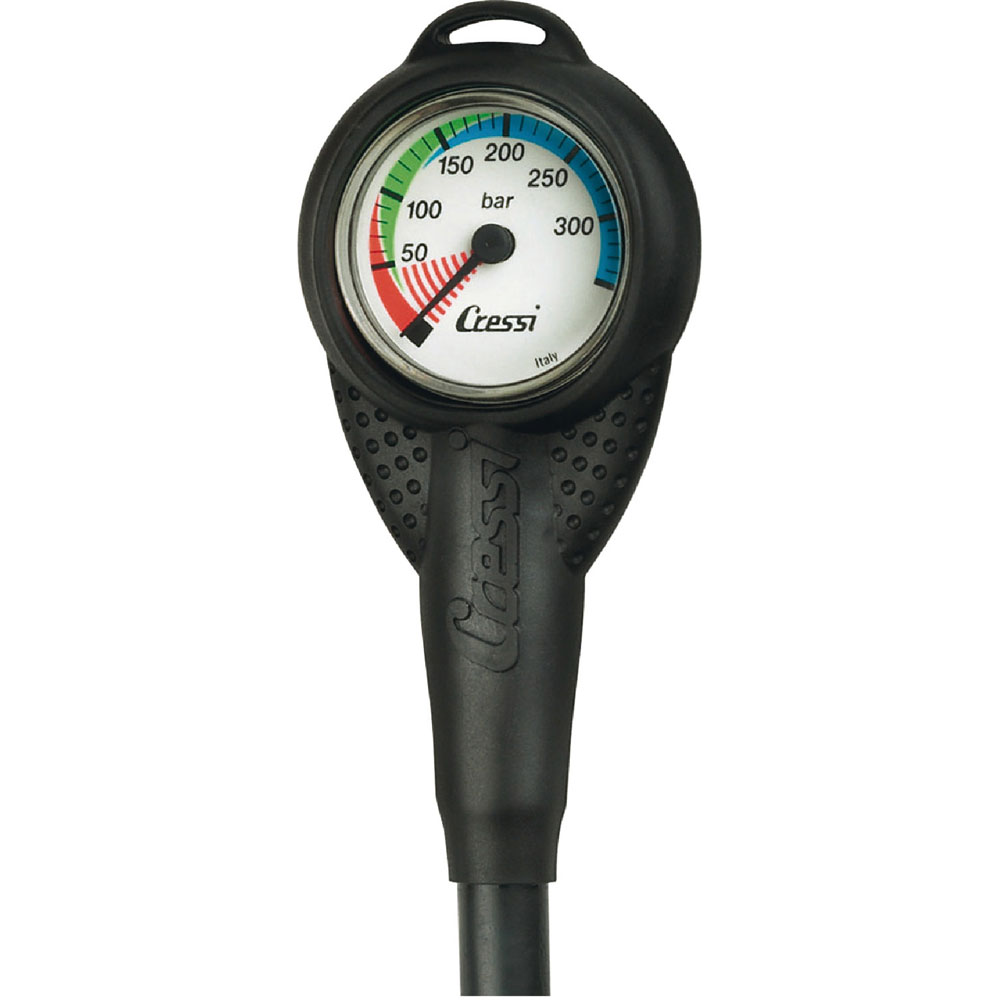The image showcases a pressure gauge designed for measuring underwater or air pressure, possibly a diving accessory given the brand. The gauge features a black, rubberized casing that narrows into a cylindrical tube at the bottom, suggesting it connects to another device. The dial is circular and encased in clear plastic or glass, displaying an arc of color-coded pressure readings. From left to right, the scale begins at 0 with a red zone extending to 50, transitions to green from 50 to 150, and then to blue ranging from 150 up to 300. The gauge also has a black hand that's currently positioned in the red section. Multiple increments mark the gauge in steps of 50, aiding precise measurement. The brand name "Cressi" is prominently molded vertically on the rubber casing and etched into the dial face along with the marking "Italy" at the bottom. The photo is taken against a plain white background, typical for product listings on retail websites.